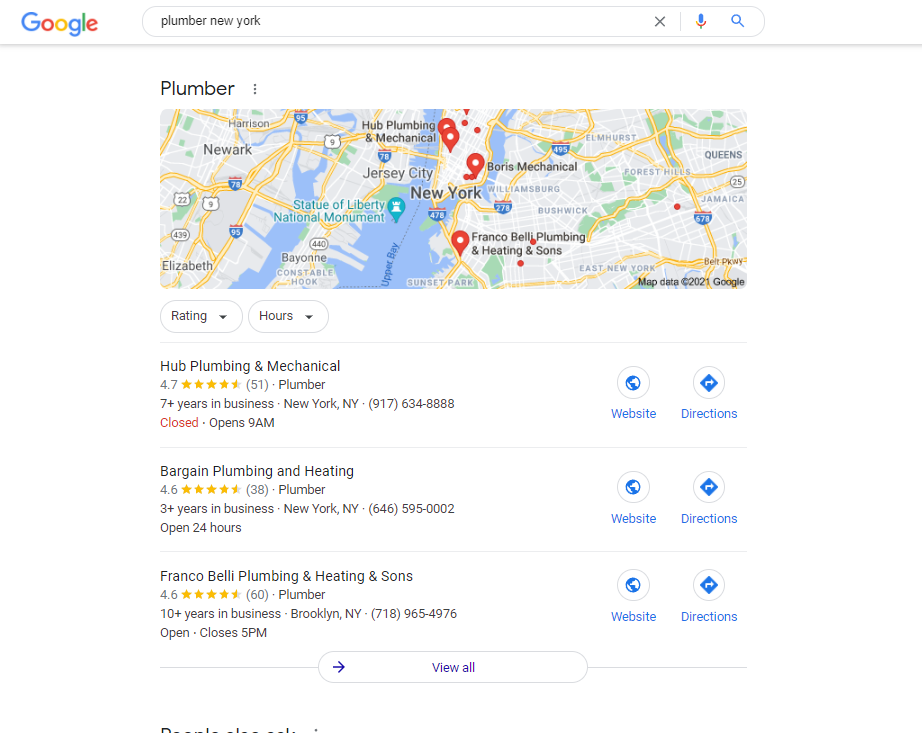The image features a screenshot of a Google search page. Prominently displayed at the top left corner is the recognizable Google logo, next to which is a search bar containing the query "Plumber, New York." Below this, a detailed map of New York and the surrounding cities, including Jersey City, Newark, and Queens, is visible. The map is dotted with pins indicating three plumbing businesses: Hub Plumbing and Mechanical, Boris Mechanical, and Franco Belli Plumbing and Heating and Sons.

Beneath the map, the details of these businesses are listed. At the top is Hub Plumbing and Mechanical, which boasts a rating of 4.5 stars from 51 reviews, is situated in New York, NY, and opens at 9 a.m. but is currently closed. It also provides a phone number and buttons for accessing the business's website and directions.

Next is Bargain Plumbing and Heating, also located in New York, NY, featuring a 4.5-star rating from 38 reviews and is notable for its 24-hour availability. This entry also includes buttons for the website and directions.

Lastly, Franco Belli Plumbing and Heating and Sons, rated at 4.6 stars, is located in Brooklyn, NY. This listing, too, is accompanied by buttons for the website and directions.